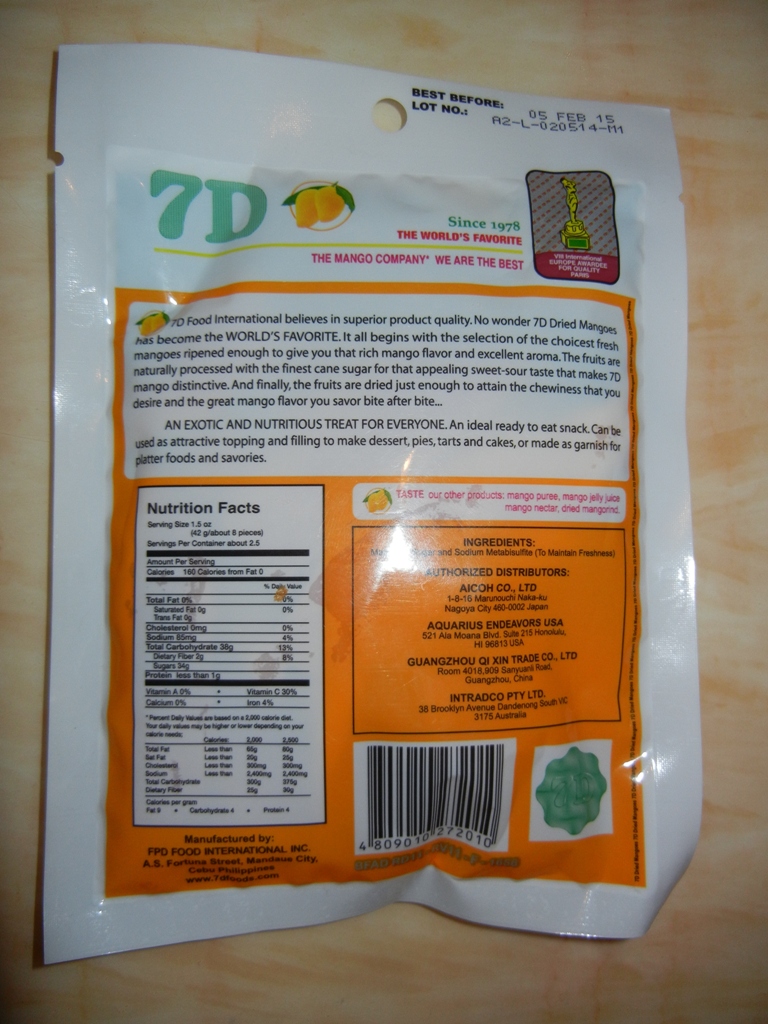The image is a color photograph of a white plastic package photographed on a marble countertop. The package features various colors and text, with a design that appears to be for dried mangoes. The prominent 7D logo at the top, displayed in turquoise, is accompanied by an image of mangoes and the text "Since 1978, The World's Favorite, The Mango Company, We Are The Best." The package also has a best-before date of 05 Feb 15, and there is a batch and lot number present. An orange-highlighted mission statement follows beneath this text. At the very top of the package, there are two slits for easy tearing, along with a circular hole for hanging. In the center, there's a highlight indicating the presence of the contents inside. The back of the package is orange with black text, a white UPC symbol, and an area detailing the nutrition facts and ingredients, along with information about authorized distributors.